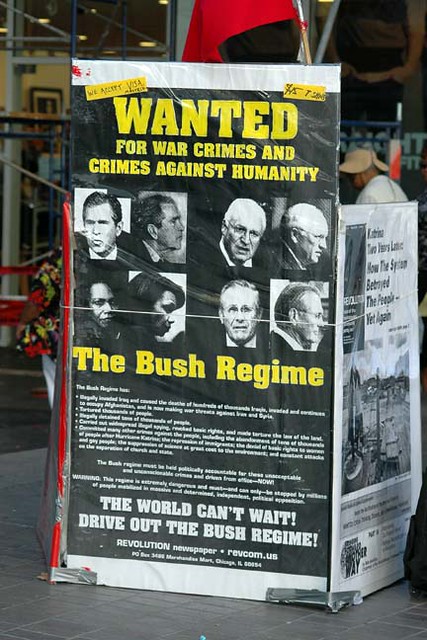The photograph depicts a politically charged poster displayed outside an uncertain establishment, possibly a cafe, with fencing in the background. The poster prominently features a headline in large, bold letters, stating "Wanted for War Crimes and Crimes Against Humanity" with the emphasis on "Wanted for War Crimes" and "The Bush Regime" in striking yellow text. The central design resembles a wanted poster, featuring black and white mugshot-like images of George W. Bush, Dick Cheney, Condoleezza Rice, and Donald Rumsfeld arranged in head-on and profile views. Below these images, there's a detailed list, though illegible in the photo, presumably outlining alleged war crimes. The lower section of the poster reads, "The World Can't Wait, Drive Out the Bush Regime," attributed to the Revolution Newspaper. Adjacent to this main poster appears to be another related political poster, hinting at the Iraq and Afghanistan Wars. Above the sign, a red flag with some white detail partially visible flutters. This scene likely dates back to the early 2000s, during a period of heightened protest against the Bush Administration's actions.